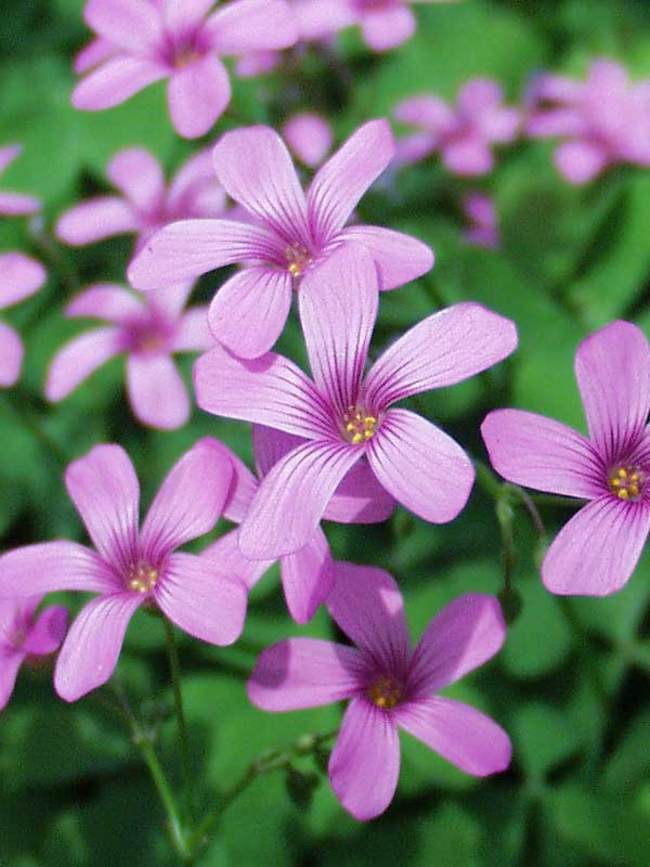A captivating photograph features a cluster of delicate purple flowers, taking center stage against a backdrop of blurred kelly green foliage. The focal point of the image is a prominent flower, displaying five distinct petals radiating from its core. The petals exhibit a gradient from an intense purple at the center to a soft, light lavender at the edges. Intricate striations add depth to the petals, further enhancing their beauty. At the heart of the central flower, tiny yellow pollen-covered stamens stand out, adding a touch of warmth to the cool hues. The soft-focus background of lush green leaves subtly frames the vibrant blooms, making them the undeniable highlight of this arresting composition.